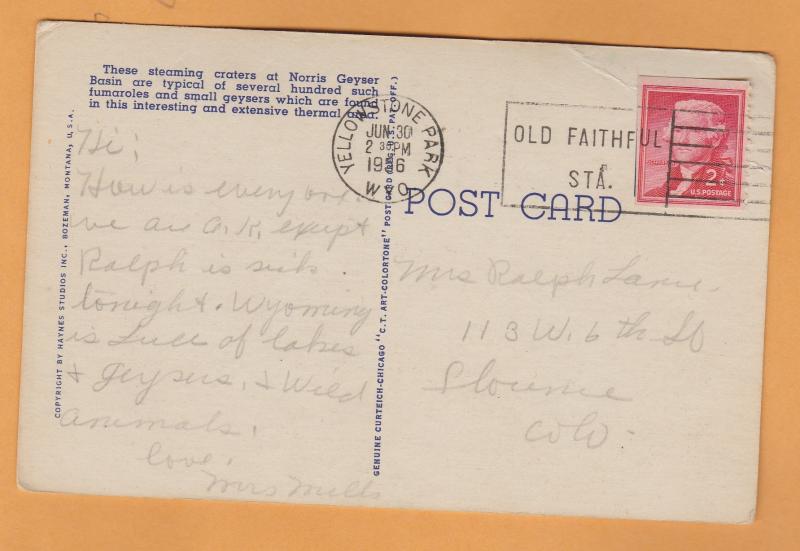The image is a photograph of the back of a white postcard, set against a light brown background. The postcard originates from Yellowstone National Park and has a date inscribed in dark blue ink: June 30th, 1936. However, the "3" in "1936" is somewhat illegible and may be another number. Prominently, the top left of the postcard features a printed caption in blue ink describing "the steaming craters at Norris Geyser Basin" as typical examples of the numerous fumaroles and small geysers in the area.

The postcard contains a handwritten note in light pencil, but the text is too faint to be read clearly. The center of the postcard is marked by a faded, Old Faithful stamp, while the right side features a red, two-cent stamp depicting a historical figure, likely an old president, potentially George Washington wearing a powdered wig. The postcard is addressed to a recipient whose details remain unreadable. This artifact, sent from Old Faithful Station, stands as a historical memento of Yellowstone's geothermal wonders.